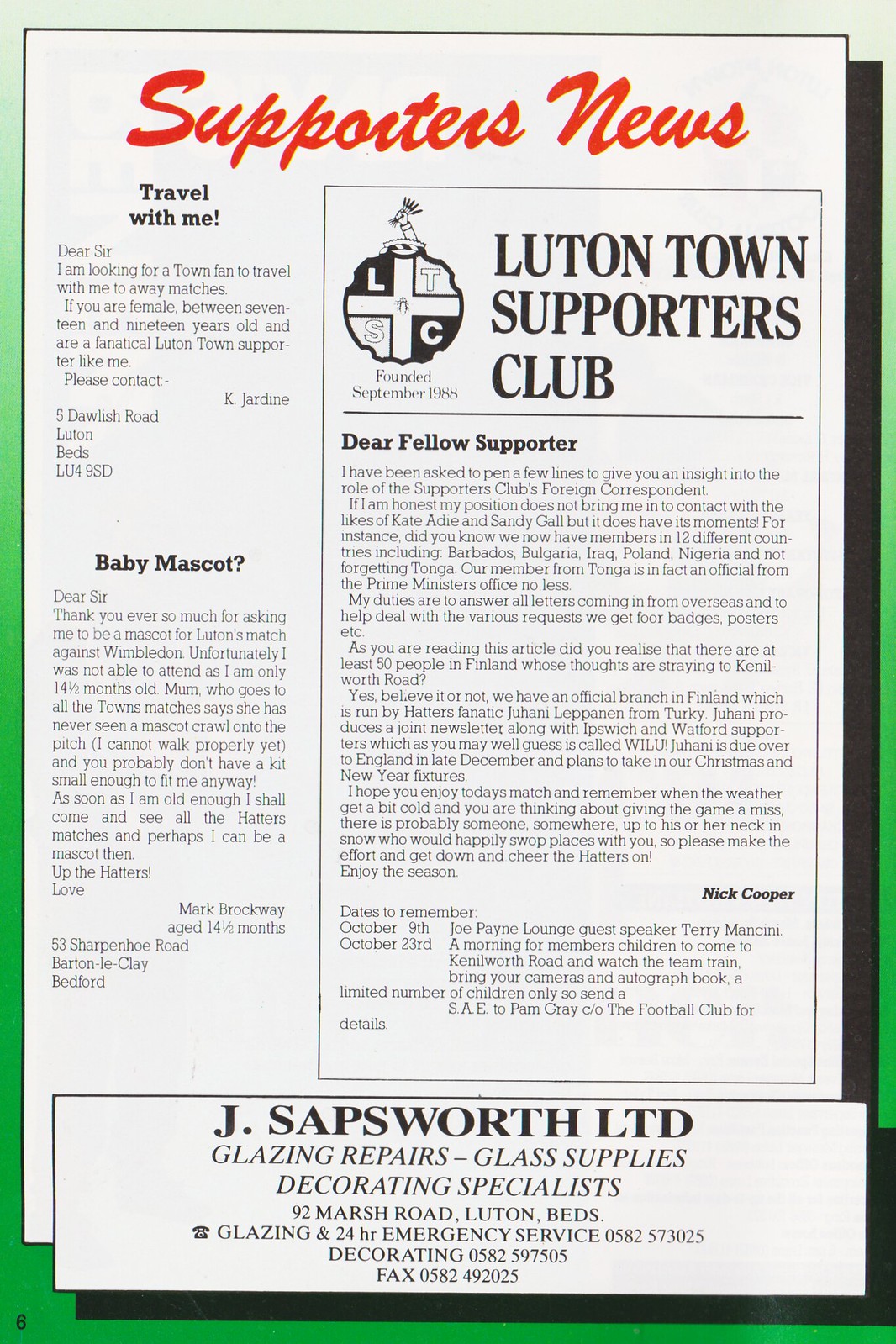The image depicts a vintage newsletter page from the Luton Town Supporters Club, framed by varying shades of green and titled "Supporters News" in red cursive at the top. Inside a white rectangle outlined in black, the left side features the headline "Travel With Me!" adjacent to the bold, capitalized "LUTON TOWN SUPPORTERS CLUB" with its logo, along with "Founded September 1988" underneath. The newsletter opens with a heartfelt message, beginning with "Dear Fellow Supporter," followed by a partially readable letter signed by Nick Cooper in bold black. Nestled on the left side is another snippet titled "Baby Mascot?"—a charming letter from an almost-15-month-old named Mark Broadway, expressing gratitude despite his inability to attend a mascot event. The bottom of the page showcases a promotional rectangle for "J.P. Sapsworth Ltd," detailing their services in "Glazing Repairs-Glass Supplies" and "Decorating Specialists," located at "92 Marsh Road, Luton, Beds," along with multiple contact numbers for their 24-hour emergency service and other business inquiries: "0582-573025" for glazing, "0582-597505" for decorating, and "0582-492025" for faxes. The overall tone of the newsletter is a blend of community engagement and practical service information, capturing the spirit and support of Luton Town's fanbase.